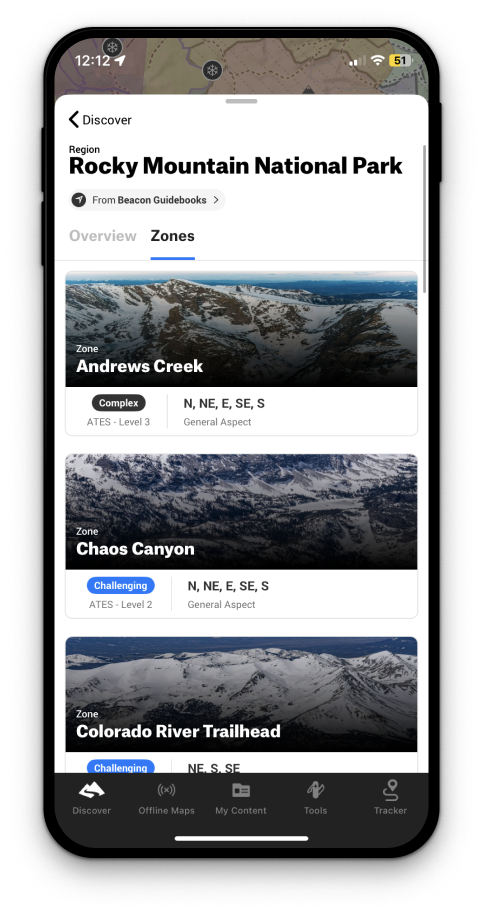A user has posted a photograph showcasing an Android phone displaying a screenshot of a map application. The screen shows detailed information about Rocky Mountain National Park, particularly focusing on different zones within the park. The current zone selected is "Andrews Creek," which is marked with a complexity level of 3. Additionally, it lists "NNESES General Aspects," though the meaning is unclear. Below "Andrews Creek," "Chaos Canyon" is visible with a challenging level of 2 and the same "NNESES General Aspects". The last visible zone is "Colorado River Trailhead," but the challenging level gets cut off and similarly lists "NNESES General Aspects." The phone interface and map details reflect intricate navigational data for visitors exploring the park.